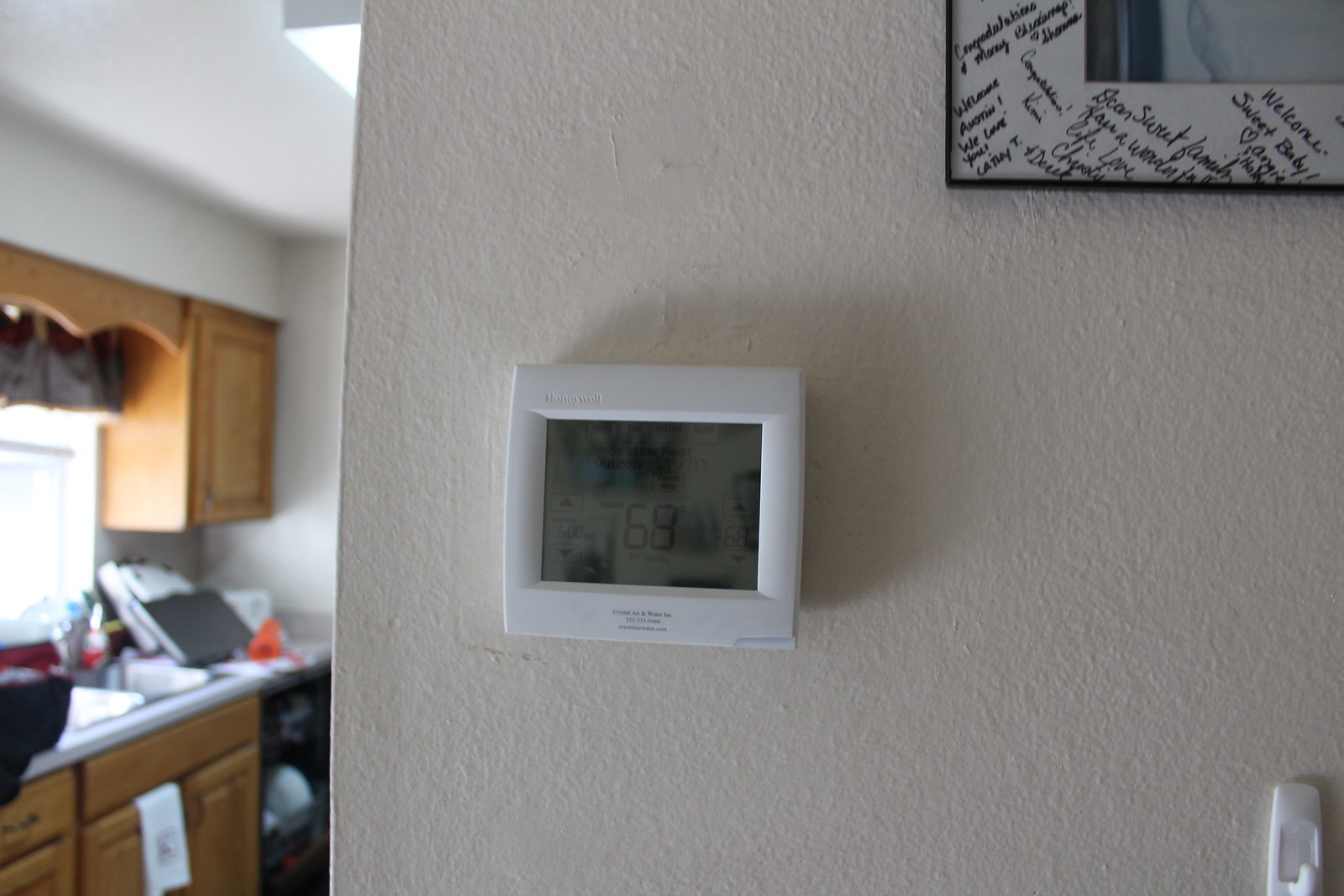The image is an indoor, close-up photograph taken in low light. Dominating the right two-thirds of the scene is a white wall, and central to this portion is a square digital thermostat with a plastic bezel and a rectangular LED display. The display shows a blurred temperature reading of 69 degrees, and any text or print on it is illegible. 

At the upper right edge of the frame, the lower left corner of a framed, multi-signed picture is partially visible. In the lower right corner, there is an empty, inexpensive plastic adhesive hook mounted on the wall.

The left third of the image provides a blurred view into a kitchen. It has wooden cabinets above and below a wooden countertop. A window at the center of the left edge lets in some light, highlighting a fluorescent light fixture on the ceiling further to the left.